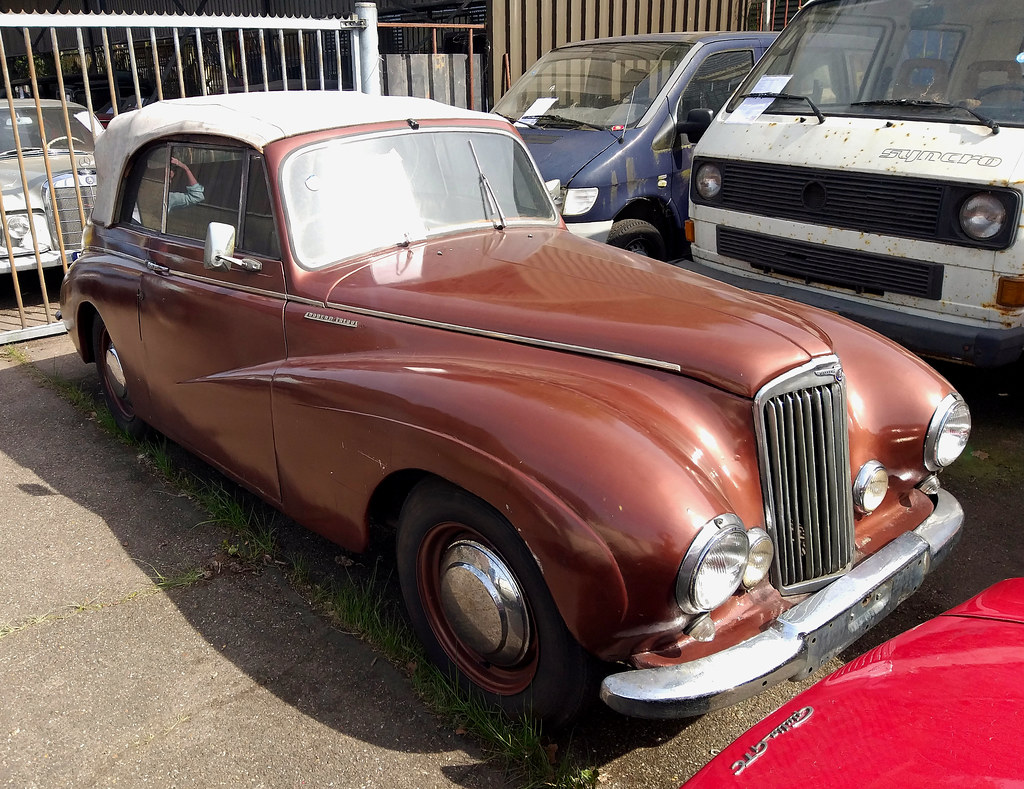The image depicts an older, possibly mid-20th-century parking lot with various aged vehicles. The centerpiece is a dark brownish-maroon car with a white roof, featuring a distinctive silver, vertically-lined grille and four headlights. Notably, the car's windshield wiper is standing straight up. The driveway is paved, though grass is emerging through the cracks. To the right of the main car is an old, broken-down white van and next to it, a similarly decrepit bluish van. In front of the main car, only the bumper of a red sports car is visible. Behind the main car, a rusted silver metal gate stands, with a brighter white section of the gate transitioning to a golden gate, next to a brown barrier. In the top right background is another vehicle, possibly a silver car from the 1950s era. In the back seat of the main car, a man in a blue shirt rests his arm, hand on forehead, contributing a lifelike element to the scene.